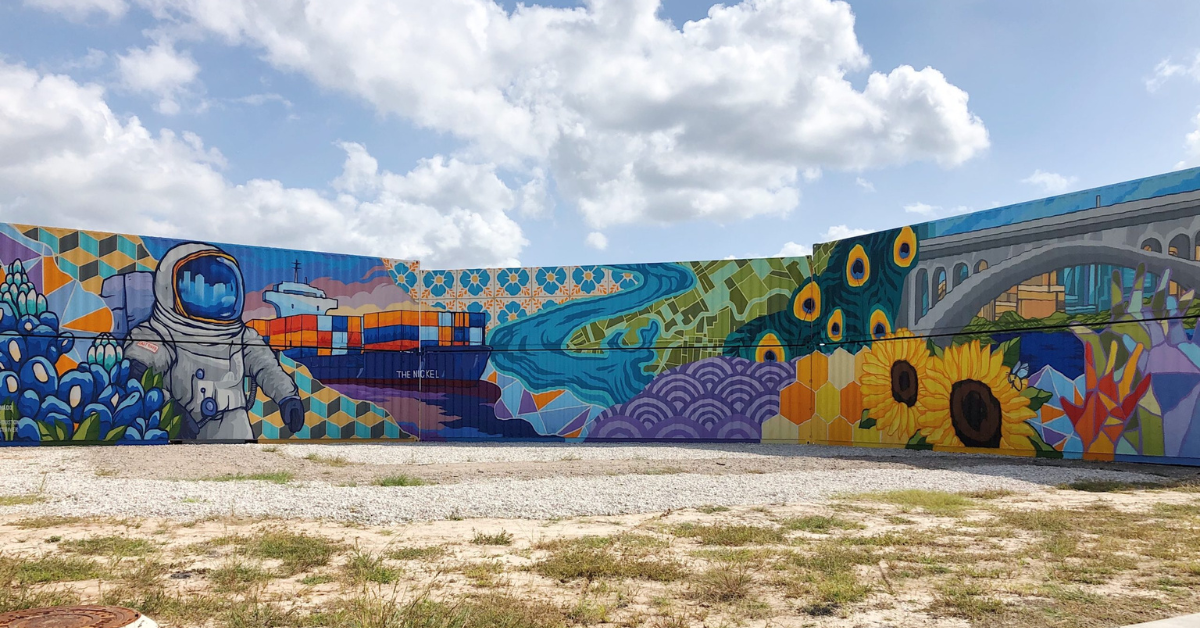The image captures a barren field with patchy grass, featuring many bald spots where the grass hasn't grown. The foreground is mainly dirt and gravel with sporadic grass tufts. Dominating the background, there are large connected walls, each adorned with vibrant and individually distinct murals. These murals showcase a variety of motifs, including a vivid blue stream flowing through purple rounded patterns, and an astronaut in a white suit with a blue mask surrounded by checkered patterns and blue flowers. One section depicts honeycombs and sunflowers—one larger than the other—while another illustrates a bridge connecting two points. The overall scene is characterized by the murals' bold colors—blues, whites, greens, yellows, purples, and oranges—against a bright, partly cloudy blue sky. Despite their individual styles, the murals blend harmoniously, enhancing the vivid ambiance of the otherwise desolate landscape.